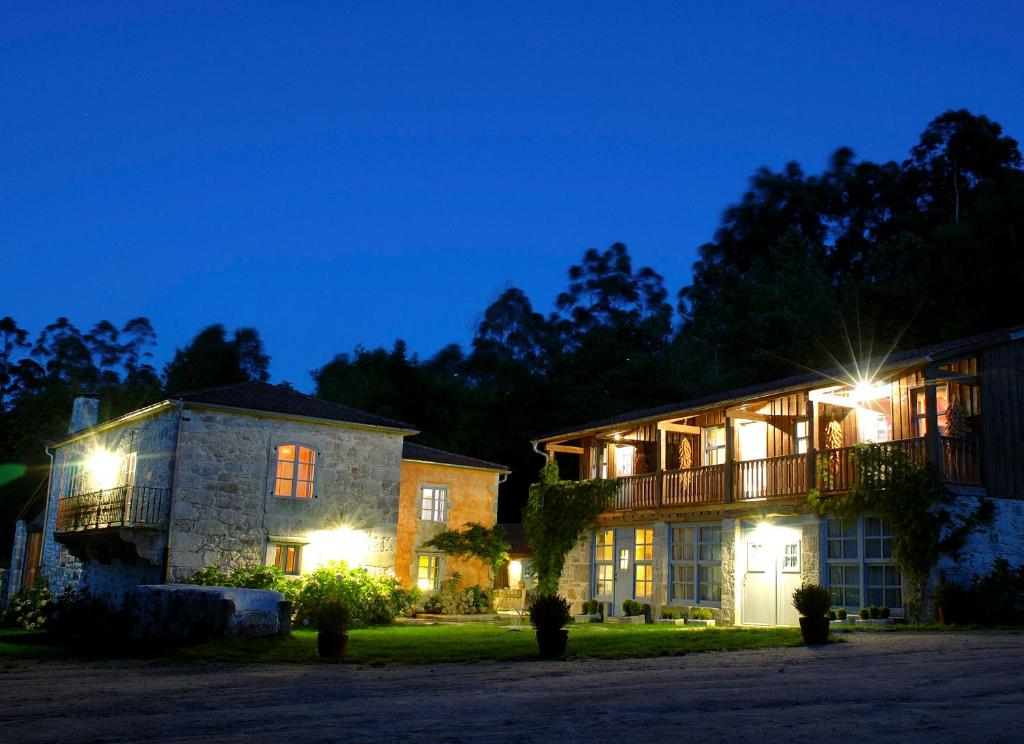This is a nighttime, photorealistic photograph of an estate featuring two distinct interconnected buildings and a separate structure off to the side. The scene is dimly lit with visible electric blue sky indicative of dusk or sundown. The building on the left is a two-story villa made of brick on its left side with a large center window, a smaller window at the bottom lined with green brush, and a veranda with a door. The bottom of this building also features a brown door surrounded by flowering bushes.

Adjacent to the villa, and seeming more modern, is a two-story extension made of reddish-brown brick and wood. This right-side building displays a series of large glass windows along its bottom floor and a wooden deck extending across the entire second level. The deck is lined with three white doors, each equipped with its own set of windows and individual lights.

The estate is framed by a yard with green grass, scattered smaller bushes, and a rectangular stone. Following this are large windows lining the base of the buildings and two main gray doors centrally situated. Additionally, trees encircle the entire complex, casting shadows over the dimly lit road out front. The whole area is alive with the glow from the lights in every room, emphasizing the estate's connection to nature and modern architecture.